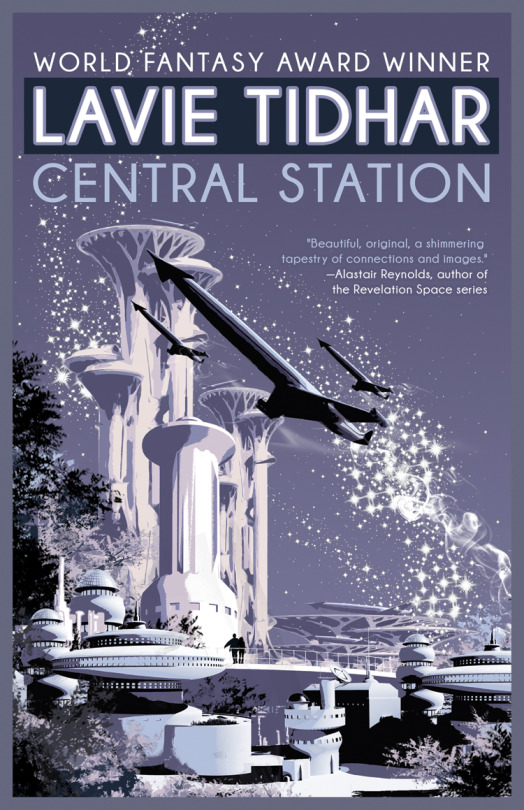The poster, framed by a dark gray background and a solid gray border, prominently displays in bold white text at the top, "World Fantasy Award winner." Beneath this, the name "Lavie Tidhar" appears in large, white, capital letters with a gray border, followed by "Central Station" in slightly smaller light blue text. The lower section features a quote, "Beautiful, original, a shimmering tapestry of connections and images." attributed to Alastair Reynolds, author of the Revelation Space series, in smaller gray font.

The visual elements of the poster highlight a starry galaxy as the backdrop, filled with fantastical and science fiction imagery. Three sleek aircraft soar through the air towards the upper left. The scene is dominated by tall, white towers resembling beakers or vases, interspersed with round and disc-shaped sci-fi buildings, set against a light purple-to-grayish purple sky. The structures vary in height and form, creating a futuristic skyline. Additionally, green trees are visible on the left, adding a touch of nature to the otherwise otherworldly setting.